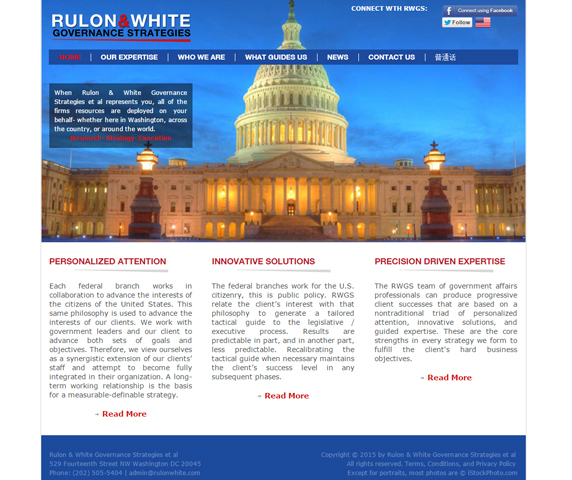This is a detailed screenshot from a website divided into two distinct sections. The top half features an image of an impressive state building resembling a palace, with two white marble floors and a massive dome capped by an unnaturally blue, dusky night sky. The website's branding is prominently displayed; in the upper left, "Rulan" is written in large white font, with the ampersand "&" highlighted in red, followed by "White" in a consistent white font. Below this, the phrase "Governance Strategies" appears in black font. 

On the upper right corner, the text "Connect with RWGS" is visible, along with interactive buttons for Facebook and Twitter, plus a small American flag icon. Directly beneath the image, a blue navigation bar contains various menu options including "Home," "Our Expertise," "Who We Are," "What Guides Us," "News," and "Contact Us." The "Home" tab is selected and indicated by a red highlight. Below the navigation bar, in a small grey rectangle, the text reads: "When Rulan & White Governance Strategies represent you, all the firm's resources are deployed on your behalf, whether here in Washington, across the country, or around the world." The bottom half of the screenshot simply has a clean white background, likely serving as a blank canvas for additional content or continuation of the page.